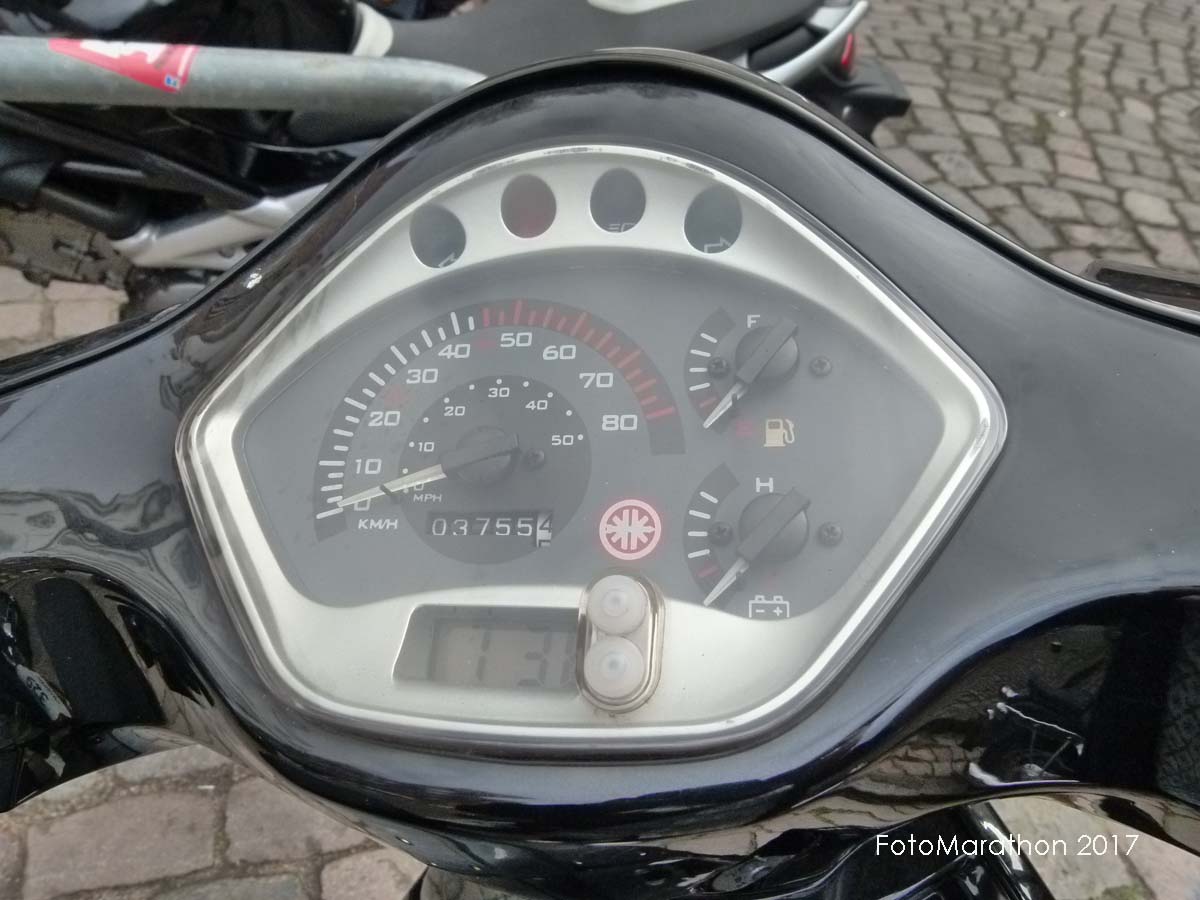The photograph captures a detailed view of the dashboard of a motorcycle, showcasing its black finish. This scene is set outdoors on a cobblestone driveway, lending a textured backdrop to the image. Prominently displayed on the bottom right corner of the dashboard is the inscription "Photo Marathon 2017." The dashboard itself features a variety of gauges and indicators: a fuel gauge is situated on the right, while the digital display reads a mileage of 3,755 miles. Additionally, the display may be showing a time of 7:38, although this detail is not entirely clear. Overall, the photograph combines elements of the motorcycle's functionality with the ambiance of an exterior setting.